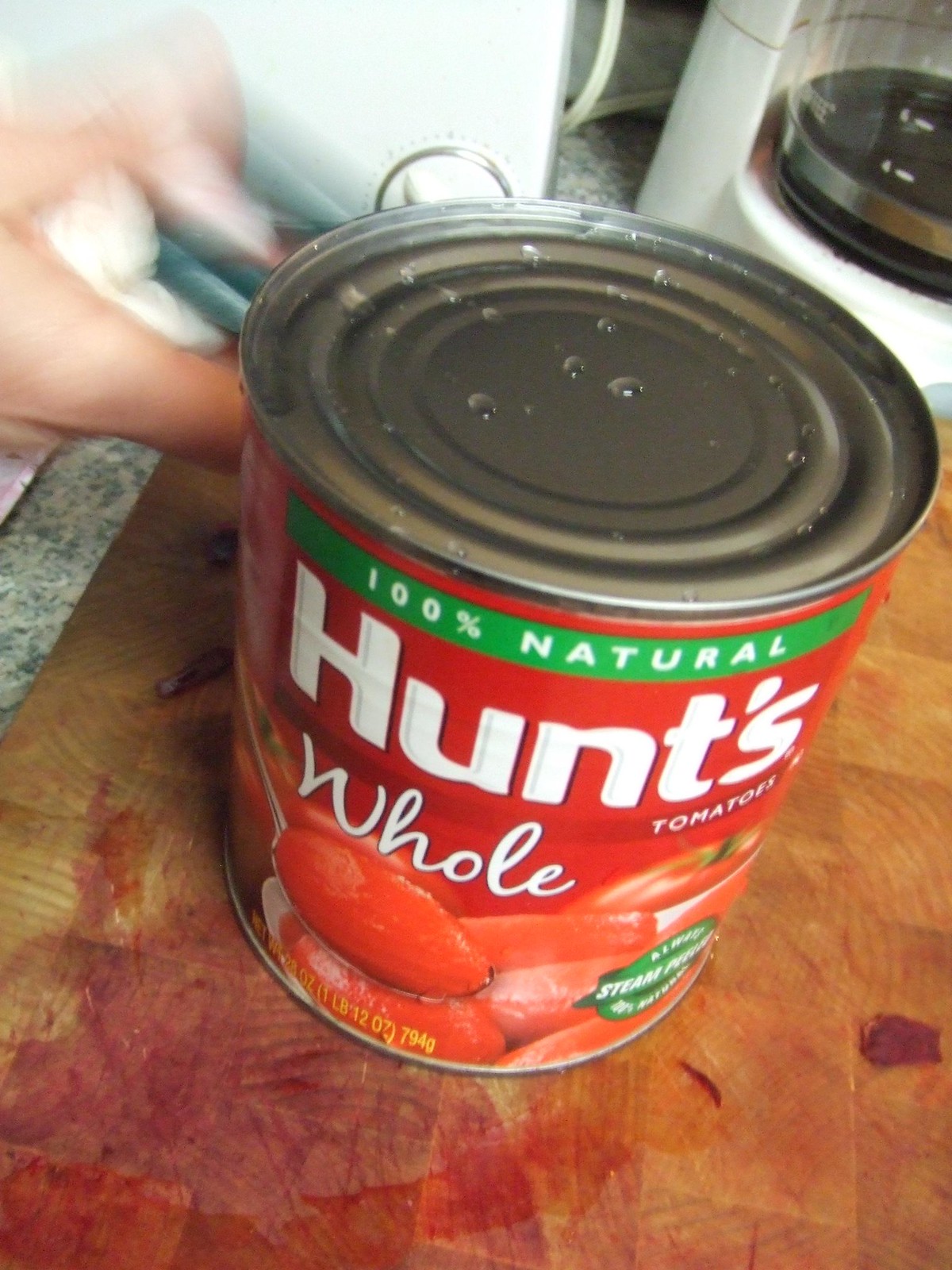This detailed image captures a kitchen scene focused on a can of Hunt's whole tomatoes placed on a wooden cutting board. The can prominently features a red label with the words "Hunt's" written in large white letters, along with "100% natural" in a green bar at the top. Below, the label also indicates "whole tomatoes" in smaller white text. The label showcases a spoon holding a tomato, surrounded by images of other tomatoes, both stacked and whole. The silver lid of the can displays water droplets, and there are visible concentric circles for texture.

The wooden cutting board, possibly a counter, shows signs of previous use with lines and a red-tinted residue. To the left, a hand with an extended index finger is lightly touching the can. In the background, a white Mr. Coffee coffee maker is visible on a granite counter, identifiable by its plastic white frame, glass coffee pot with a silver band, and white markings indicating coffee levels. A white cable and another white appliance featuring a knob are also partially visible in the upper left section of the image.